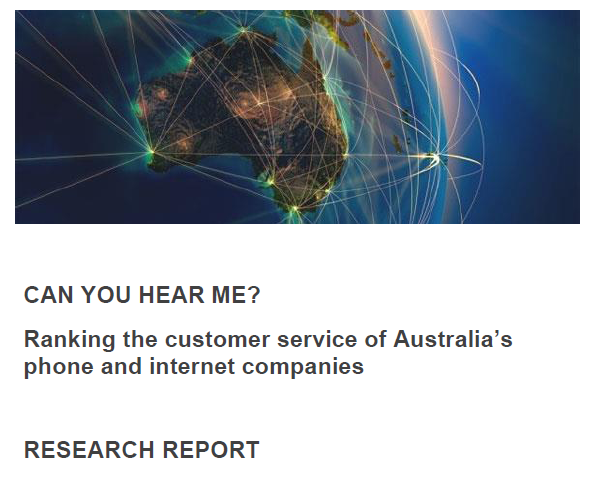The image depicts a visually striking representation of Australia at the top, possibly digitally rendered, showcasing the country's outline with a noticeable curvature of the Earth's surface. Radiating from Australia, various colored lines—pink, blue, green, yellow, and white—extend to different parts of a stylized globe, indicating communication or connectivity links. Some recognizable landforms, like New Zealand, are visible amidst the abstract geography. The upper section of the image prominently features the text, "Can you hear me?" followed by a question mark. Below this phrase, the image caption reads, "Ranking the customer service of Australia's phone and internet companies." In the bottom left-hand corner, in bold, all-capital letters and black font, the label "RESEARCH REPORT" is clearly displayed.